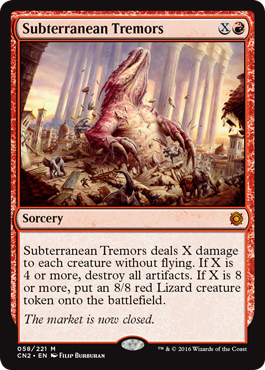This image features the Magic: The Gathering card "Subterranean Tremors," a card from the acclaimed collectible card game produced by Wizards of the Coast, a subsidiary of Hasbro. Wizards of the Coast is also known for Dungeons & Dragons, and the mutual influence between these two games is evident. 

In this specific card, players will recognize its affiliation with the red color mana, crucial for a deck centered around red strategies. Magic: The Gathering features five colors—red, white, blue, green, and black—and although cards can feature combinations of these colors, "Subterranean Tremors" is purely red.

The name of the card is prominently displayed at the top, accompanied by a unique mana cost symbol — an "X" in a circle next to a red symbol, indicating that players must pay one red mana in addition to any amount of other mana. The card's artwork dramatically captures a colossal creature erupting from the ground, forcefully scattering elephants to illustrate its immense power.

Below the illustration, the card type is labeled "Sorcery," and its specific abilities are detailed further:

"Subterranean Tremors deals X damage to each creature without flying. If X is four or more, destroy all artifacts. If X is eight or more, put an 8/8 red Lizard creature token onto the battlefield."

Adding a touch of humor, the card includes flavor text: "The market is closed."

As noted by the symbol at the bottom left corner, this card's rarity is denoted by an "M," signifying it as a Mythic rare card—highly coveted and difficult to obtain from a booster pack.

Overall, "Subterranean Tremors" is a powerful and rare addition to any red-focused Magic: The Gathering deck, offering significant tactical advantages depending on the amount of mana invested into its casting.